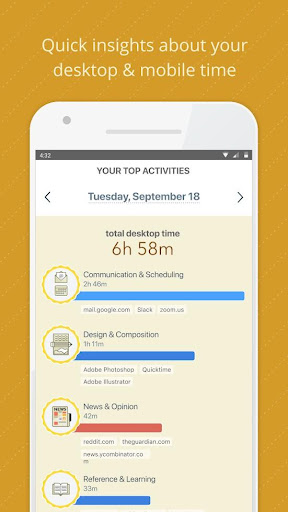The image features a detailed dashboard with an orange background. The edges are adorned with a series of dashed lines. The main content is organized into different sections, each highlighting specific activities on a desktop and mobile setup. 

At the top left, there's a gray circle indicating a presumed 4:32 time, with a partial WiFi signal and a nearly depleted battery icon next to it. Below, a smartphone swipe gesture is depicted. The dashboard also includes a timeline indicating that the top activity can be scrolled left or right.

The date displayed is Tuesday, December 18th. The total desktop usage time is recorded as 6 hours and 58 minutes, broken down into various categories:

1. **Communication & Scheduling:** Represented by a yellow circle on the left, this includes emails and meetings, specifically through platforms like Mail (mail.google.com), Slack, and Zoom (zoom.us).

2. **Design & Composition:** This section records 1 hour and 11 minutes of desktop usage, visualized by a blue bar and featuring software such as Adobe Photoshop, QuickTime, and Adobe Illustrator.

3. **News:** This category, marked by a red bar, includes sites like Reddit.com and TheGuardian.com.

4. **Reference & Learning:** Totals 30 minutes, represented with a blue bar.

The edges around the dashboard are gray, and the background color is a shade of yellow.

Overall, the dashboard offers a comprehensive and detailed breakdown of desktop usage, neatly categorized and easy to interpret.